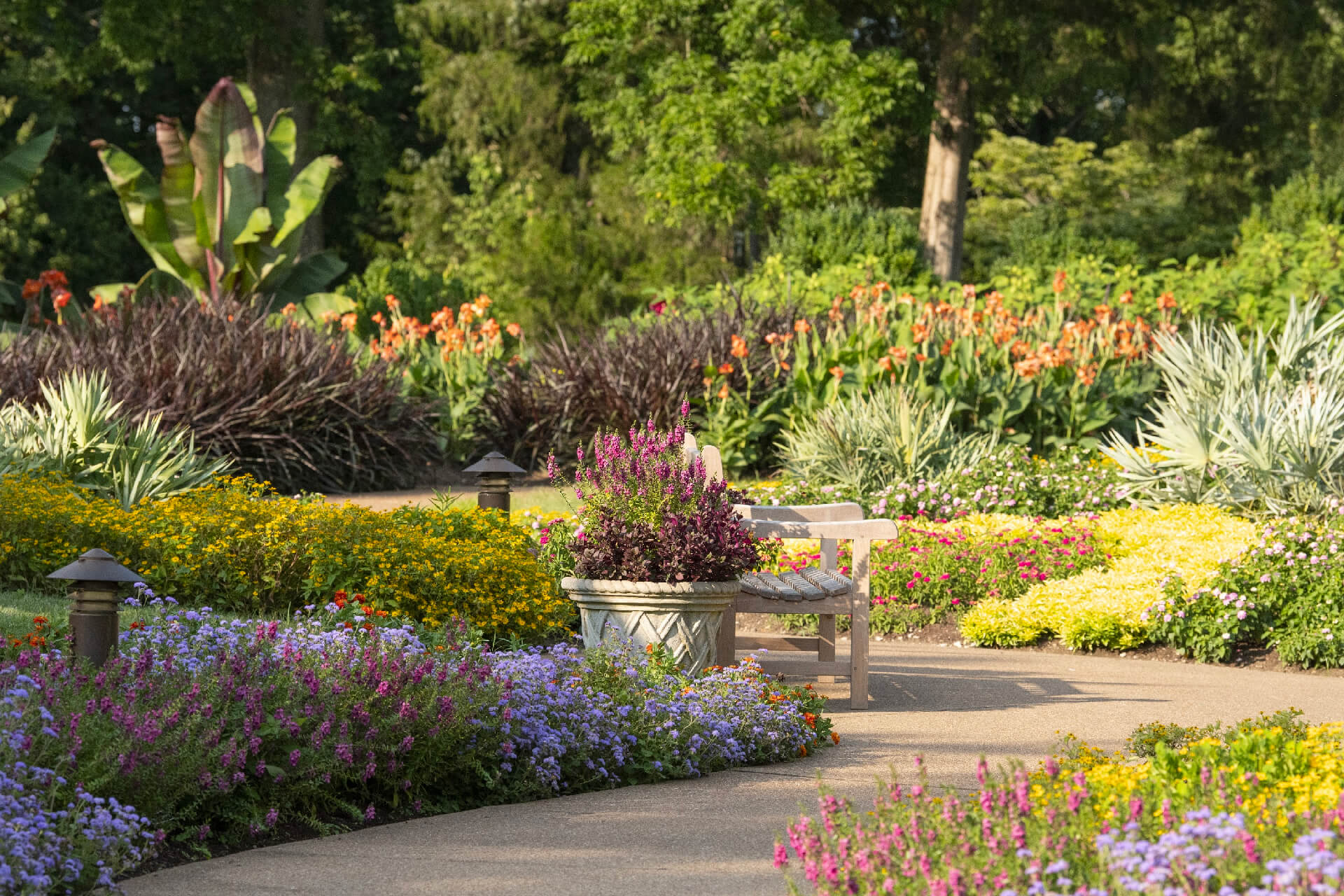This photograph captures a meticulously maintained public garden or botanical park. Prominently featured is a cement walking path originating from the bottom left corner, guiding the viewer's eye toward a white wooden bench. Flanking the bench is a large cement planter teeming with greenery, adding depth to the scene. The garden is a burst of vibrant colors, showcasing an impressive array of multi-colored flowers including purples, lavenders, pinks, yellows, oranges, and magentas, reflecting its diversity and well-kept nature. The rich hues of the flowers are matched by the fresh, vibrant greens of the surrounding bushes and plants. In the background, shadowy trees frame the garden, hinting at a more wooded area beyond. This lush, colorful setting embodies a serene and picturesque outdoor environment.